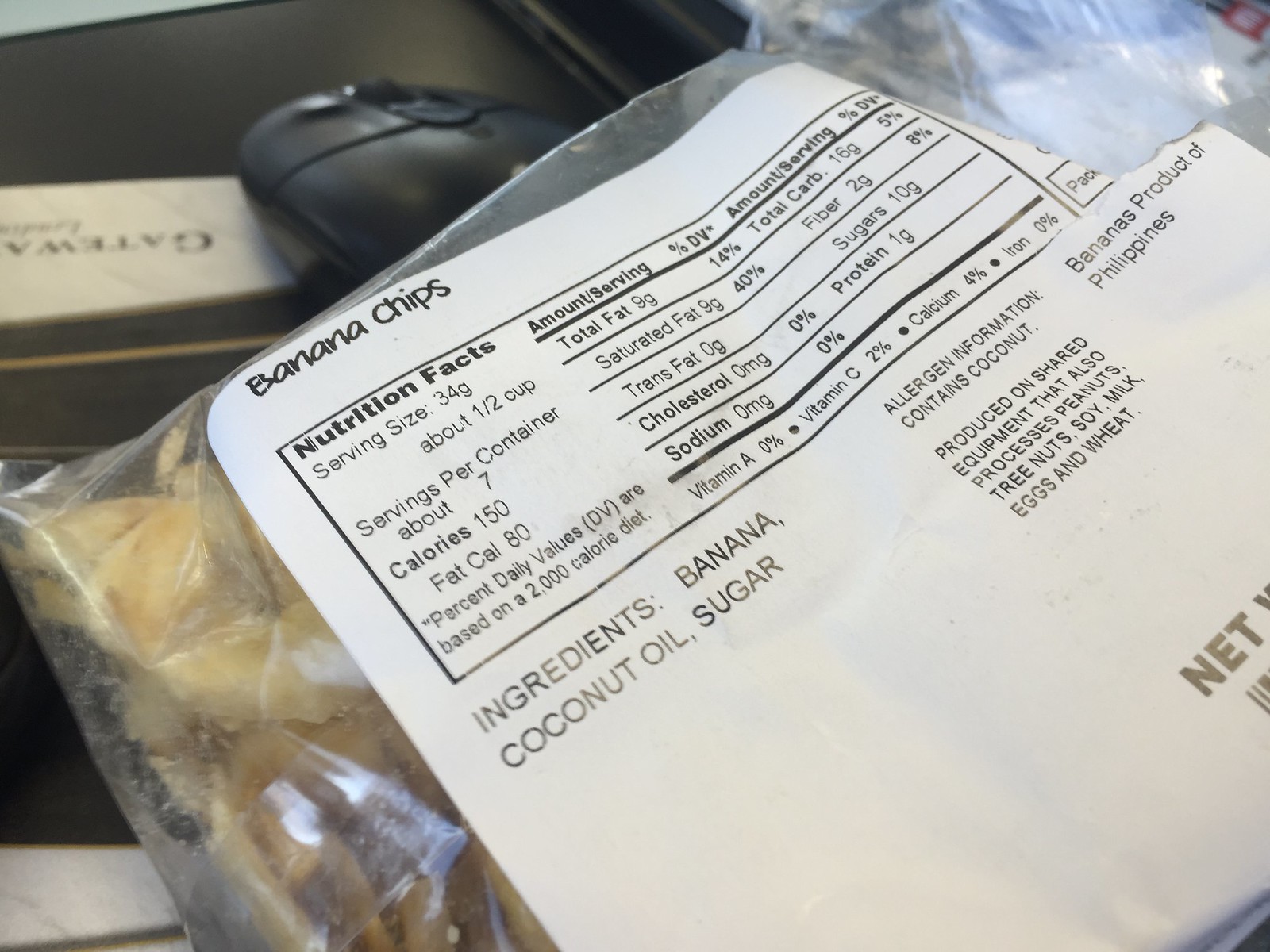This photograph, taken indoors in what appears to be a home or office setting, captures a close-up shot of a clear plastic bag from a manufacturer. A white label is adhered to the bag, prominently displaying the product name "Banana Chips" at the top. Below the title is a detailed chart with nutritional facts: a serving size of 34 grams (about half a cup), with approximately 7 servings per container. Each serving provides 150 calories, 80 of which are from fat. The ingredients list reads: banana, coconut oil, and sugar. A note indicates that the bananas are a product of the Philippines, and allergen information specifies the presence of coconut. In the background, slightly out of focus, a black computer mouse and a piece of white paper with reversed, partially visible text can be seen, adding context to the indoor environment.